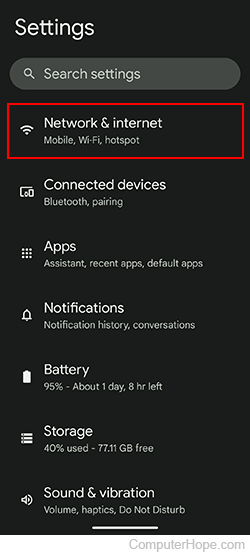The image depicts a digital settings menu interface with a sleek, user-friendly design. At the top, there's a long, black rectangular bar featuring the word "Settings" in bold, white lettering. Below this, a gray rectangle with rounded edges contains the text "Search settings" in a whitish color, accompanied by a magnifying glass icon on its left.

Beneath the search bar, a hierarchical list of settings options is displayed. The first section is enclosed in a red rectangle with a black background. It reads "Network & Internet" in white letters, under which "Mobile, Wi-Fi, hotspot" are listed.

Following this, the "Connected Devices" section includes "Bluetooth, pairing" details. Next is the "Apps" category, listing "Assistant, recent apps, default apps," and is marked with an icon of nine dots to its left.

The "Notifications" section, denoted by a bell icon, covers "Notification history, conversations." This is followed by the "Battery" section, displaying a white upward-pointing battery icon with a status of "95% - about 1 day, 8 hours left."

The "Storage" section, characterized by an icon of three lines, shows "40% used, 77.11 GB free.” Finally, the "Sound & Vibration" section, indicated by a speaker icon, includes "Volume, haptics, Do Not Disturb."

All text within the interface is presented in clean, white lettering, ensuring ease of readability against the various background colors.